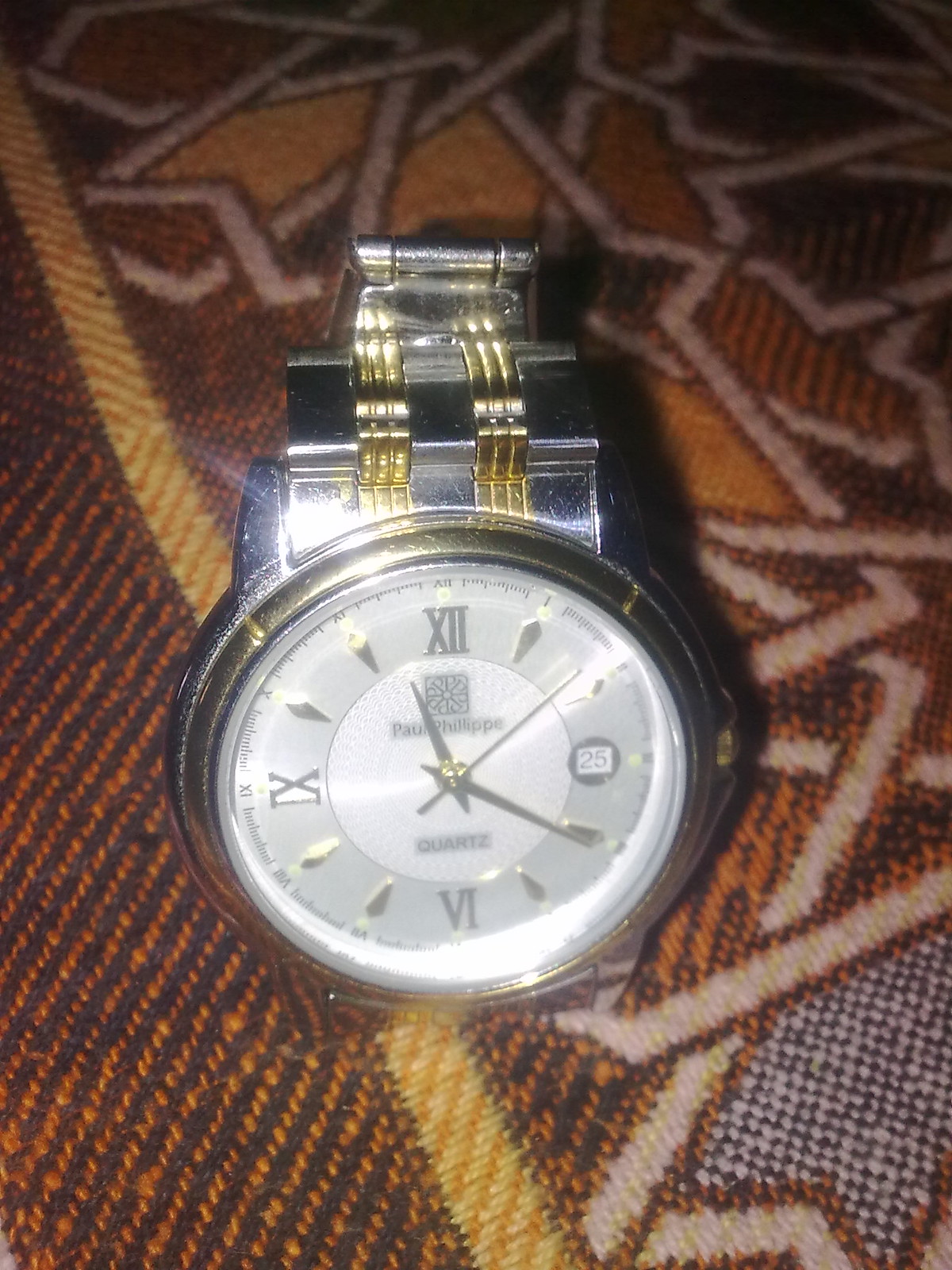The image features a silver men's watch prominently resting on a textured surface that resembles a woven carpet or canvas placemat, adorned in shades of orange, black, and tan. The watch, likely made from stainless steel, showcases a sophisticated blend of silver and gold accents. The watch band features two gold-toned stripes that extend from the face toward the links, which are primarily silver metallic. 

The circular watch face is encircled by a sturdy gold rim, and the glass appears to be heavy-duty. The background of the clock face itself is white, while it hosts three Roman numerals marking 12, 6, and 9 o'clock. Notably, the position where the 3 would typically be is replaced by a date marker displaying the number 25, suggesting the date the picture was taken. The remaining hour markers are depicted by gold-toned tick marks or small diamonds. 

Additionally, the watch contains gold-toned hour, minute, and second hands, with a quartz label positioned below them. The brand name "Paul Philippe" accompanied by a tiny square logo, is located just above the hands, adding a touch of elegance to the timepiece. Overall, the watch stands out distinctly against the intricately patterned, carpet-like background, highlighting its detailed craftsmanship.